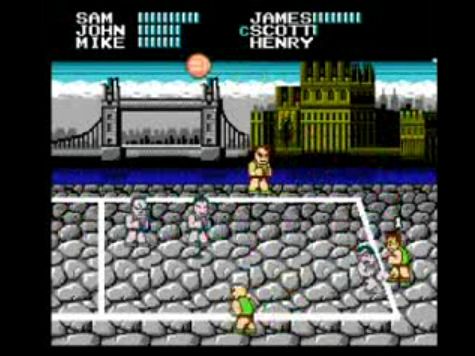A nostalgic screenshot of "Super Dodgeball" on the NES, the American version of the popular Kunio-kun series game. The image showcases the vibrant and action-packed gameplay, where players control characters using the same engine as the iconic beat-em-up games in the Kunio-kun franchise. In this fast-paced dodgeball match, players punch and throw the ball to eliminate opponents on the other side, capturing the essence of classic 8-bit sports-action games.